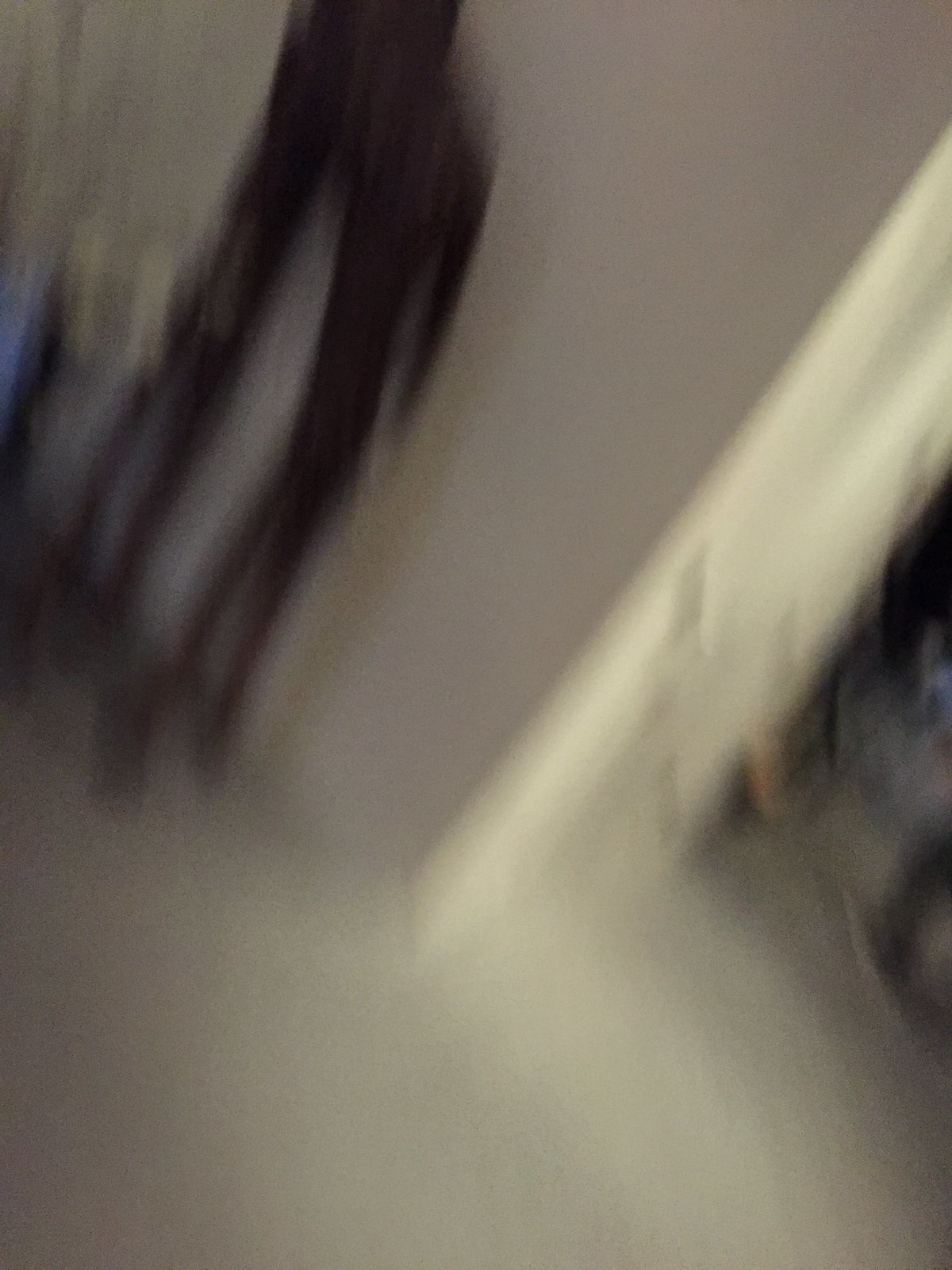This image is a highly out-of-focus photograph taken indoors, and its contents are difficult to discern due to the extreme blurriness. The photo appears to be captured at an angle from the lower center, leading up to an indistinct light-colored edge or line that stretches towards the upper right-hand corner. Above this line, there is a predominantly gray area, contrasted by a white area below it that includes some irregular dark sections on the far right-hand side. These dark sections consist of rounded, non-uniform blurs that add mystery to the setting. In the upper left-hand corner, there are two irregular black lines reminiscent of a pair of pants or giraffe-like legs, though their exact nature is unclear, and they might suggest a coat stand or other tall objects. Additionally, there is a small blue blur along the far left edge. The foreground features a smooth taupe surface. Despite the presence of these elements, the overall scene remains ambiguous, offering little context or detail to clearly identify specific objects or the nature of the room itself.